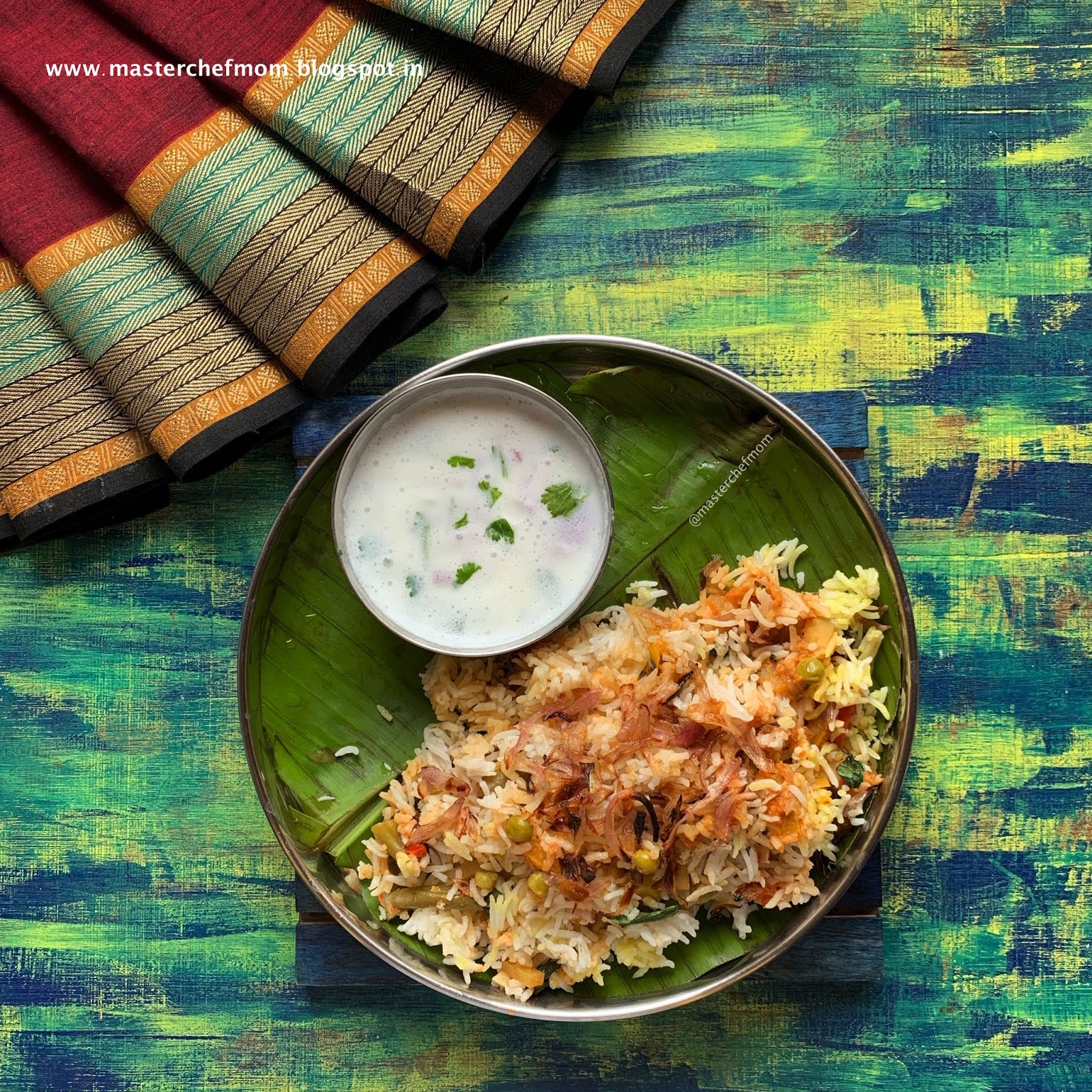The image displays an overhead view of a circular silver plate situated on a vibrantly painted wooden surface with green, blue, and yellow hues. To the upper left corner of the photo, there are vibrant, rolled napkins adorned with red, gold, and green decorations. The plate itself is divided into two sections: one side contains a mix of rice and vegetables, while the other holds a small circular bowl with a creamy white sauce topped with green herbs. Additionally, near the top left of the plate, the text "www.masterchefmom.blogspot.in" appears in white lettering, and toward the center top right corner, there's a watermark indicating "At Master Chef Mom."